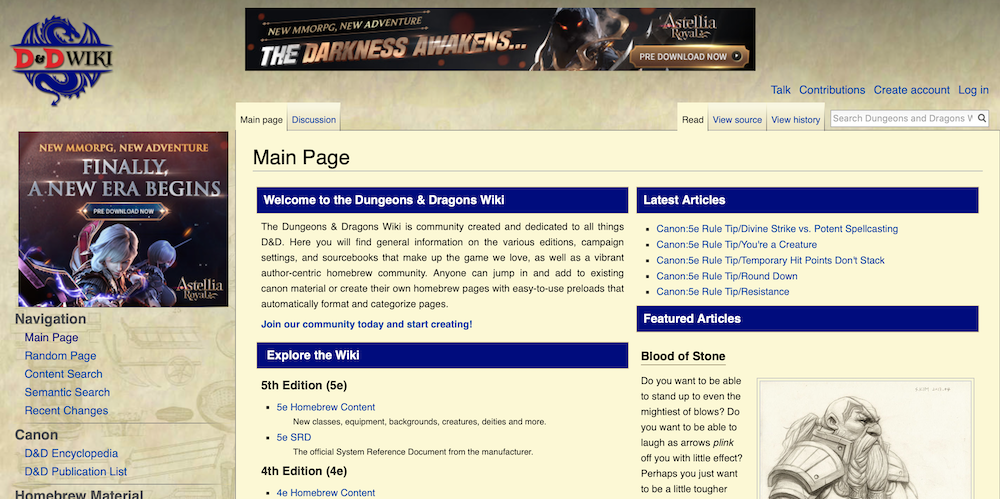This screenshot is from a webpage featuring a light beige background. At the top, there is a darker beige bar adorned with faint, hard-to-see graphics in gray. In the upper left corner, an icon of a blue dragon with wings is displayed, with the text "D&D" in red font running through the center of the dragon, followed by "wiki" in blue font.

At the top of the page, a banner advertisement reads, "The Darkness Awaits - Download Now." Below the dragon icon, another advertisement proclaims, "Finally, a New Era Begins - Aurelia - Download Now." 

Underneath this ad, a section labeled "Navigation" appears. The headings in blue font include: "Main Page," "Random Page," "Content Search," "Semantic Search," and "Recent Changes." In black font, additional links are labeled "Canon," "D&D Encyclopedia," and "D&D Publication List."

On the right side of the page, a section titled "Main Page" is evident. This section welcomes users to the "Dungeons and Dragons Wiki," describing it as a community-created resource dedicated to all things D&D.